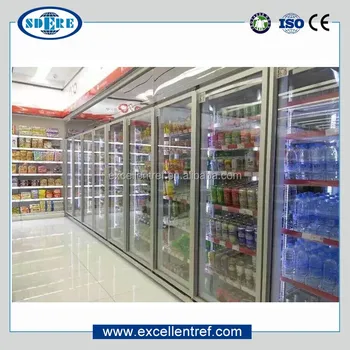This image depicts the interior of a refrigerated section in a grocery or convenience store. The foreground features a cold storage unit containing a variety of drinks, including visible bottles of mineral water and cans that could be either beer or soft drinks. The back of the section showcases shelves lined with various food items, potentially cereals or canned goods, though they are too distant to discern clearly. Fluorescent lighting illuminates the space. Notable symbols include a circular logo with the letters "STERE" in the top left corner of the image and the logos "ISO" and "CE" in the top right corner, with a third, less distinguishable symbol. At the bottom middle, the website "www.excellentref.com" is prominently displayed.